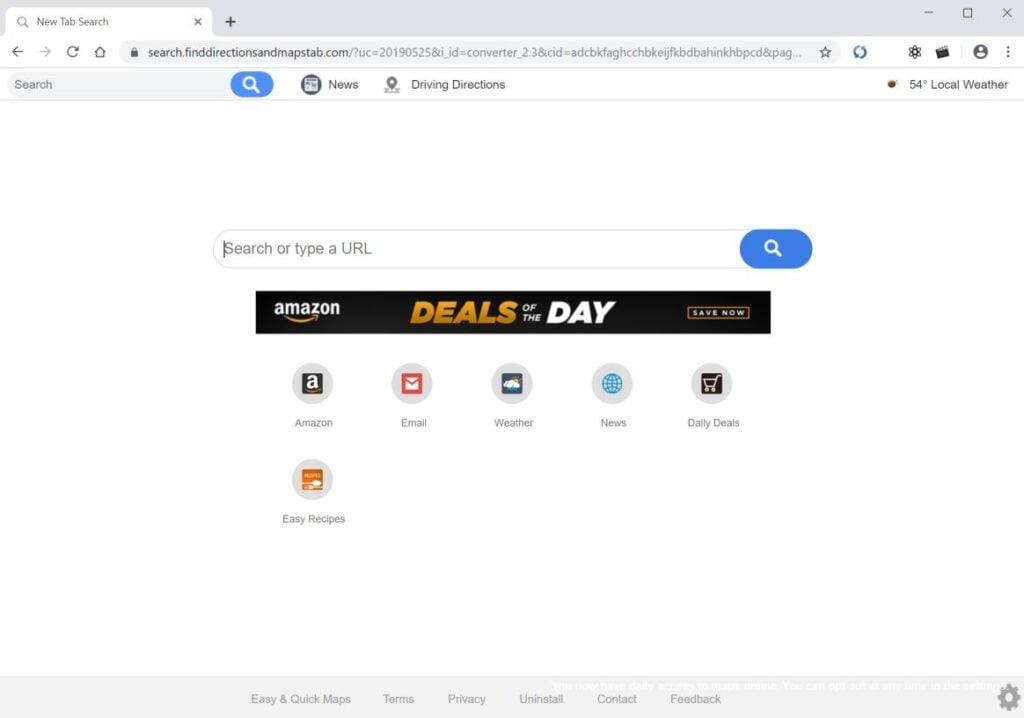A browser window is open on a "Find Directions" map tab, offering a comprehensive view packed with various navigational and search features. At the very top, a tab labeled "New Tab Search" is visible, indicating the webpage in focus. Directly below this, the familiar interface elements of a Windows search bar are lined up: a home icon, a refresh icon, backward and forward navigation buttons, and an ellipsis (three dots) button for additional options.

Below this primary window bar lies a second search bar, emphasizing the website's focus on facilitating comprehensive searches. To the immediate right of this second search bar are icons labeled "News" and "Driving Directions," providing quick access to these functionalities. On the far-right end of the search bar, a local weather widget displays the current temperature and weather conditions for the user's location.

Dominating the main body of the website is a prominent Amazon banner ad. It announces "Amazon Deals of the Day, Save Now" and features various clickable categories linked to the day's highlighted deals.